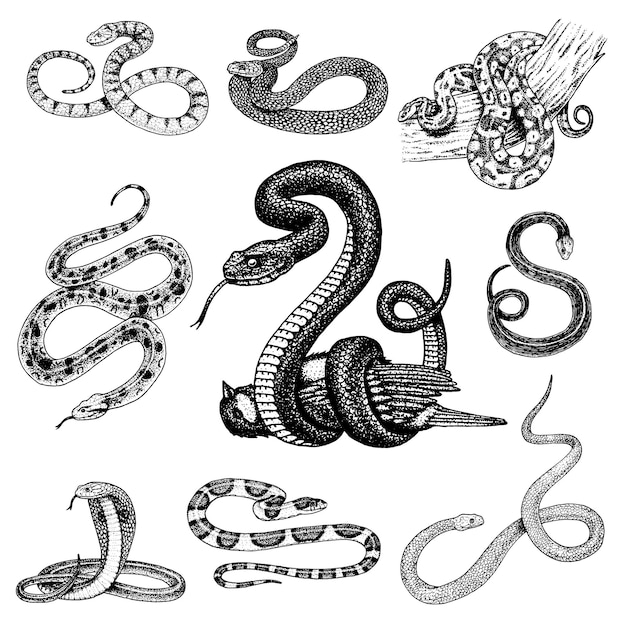This black and white pen and ink illustration depicts nine different species of snakes arranged in a 3x3 grid. Each snake is intricately detailed, showcasing various coiled positions, from S-shapes to circles. The focal point is the large snake in the center, which is more menacing than the others, with a white underbelly and its tongue sticking out. This snake is coiled tightly around a fairly large bird with a white belly and white beneath its eyes, appearing to suffocate it. Surrounding this central scene are eight other snakes. On the lower left, a cobra is distinctly recognizable by its hood. The snake in the lower middle has shiny, large black splotches. The top right features a constrictor, heavily coiled on a tree branch. Another snake, potentially a rattlesnake with diamond-shaped markings, is coiled like the cobra. Each snake varies in pattern and size, emphasizing the diversity among the species depicted.